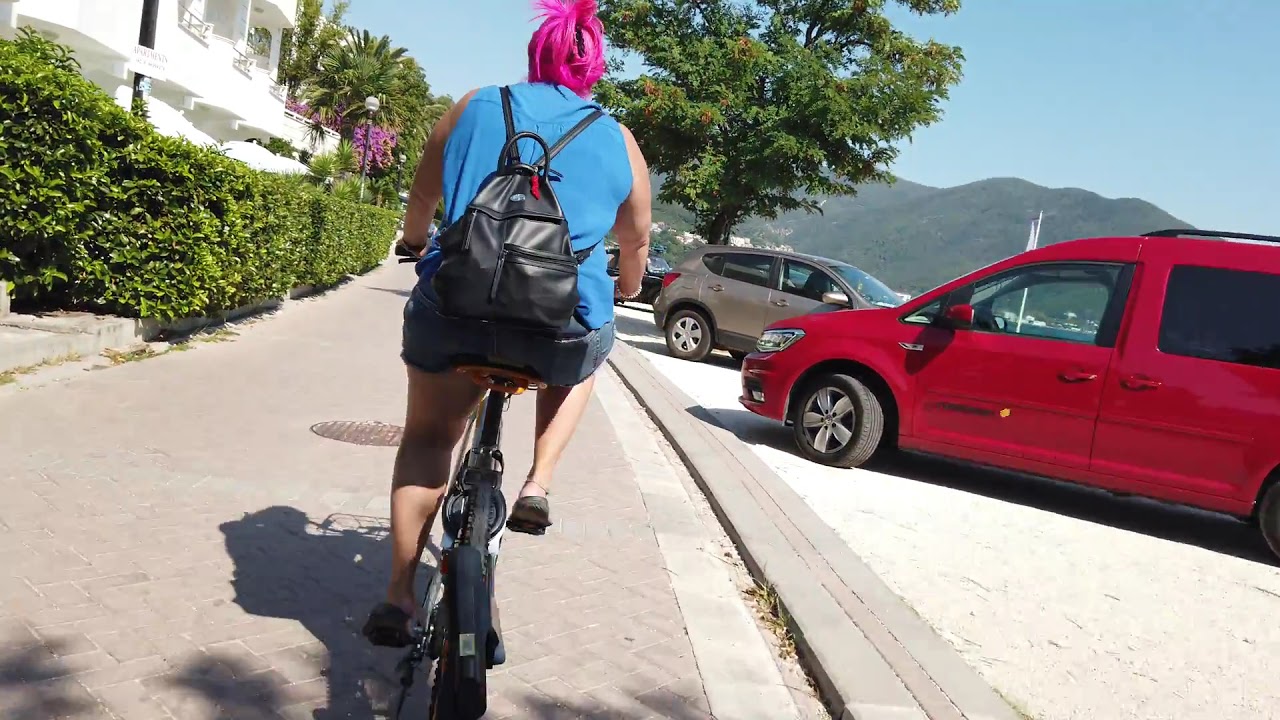The image depicts a vibrant outdoor scene, likely captured in the summertime or a warmer climate. Dominating the center is a brick sidewalk that extends from the foreground into the distance. Riding away from us on the sidewalk is a bicyclist, presumably a woman, identifiable by her blue tank top, black leather-style backpack, and bright pink hair tied into a ponytail. Her shadow stretches out beside her on the sidewalk, adding to the sunlit atmosphere.

To the left of the sidewalk, neatly trimmed hedges border what appears to be a residential building, possibly a home or condo with a balcony. Palm trees rise behind a street post on this side, accentuating the warm, possibly tropical setting. 

On the right side, an angled parking lot features several vehicles, including a red minivan parked head-in and a Hyundai SUV backed into its spot. Beyond the parked vehicles, a large tree adds a touch of greenery. In the far distance, rolling hills or mountains and a clear blue sky with no clouds are visible, completing the serene and picturesque outdoor scene.